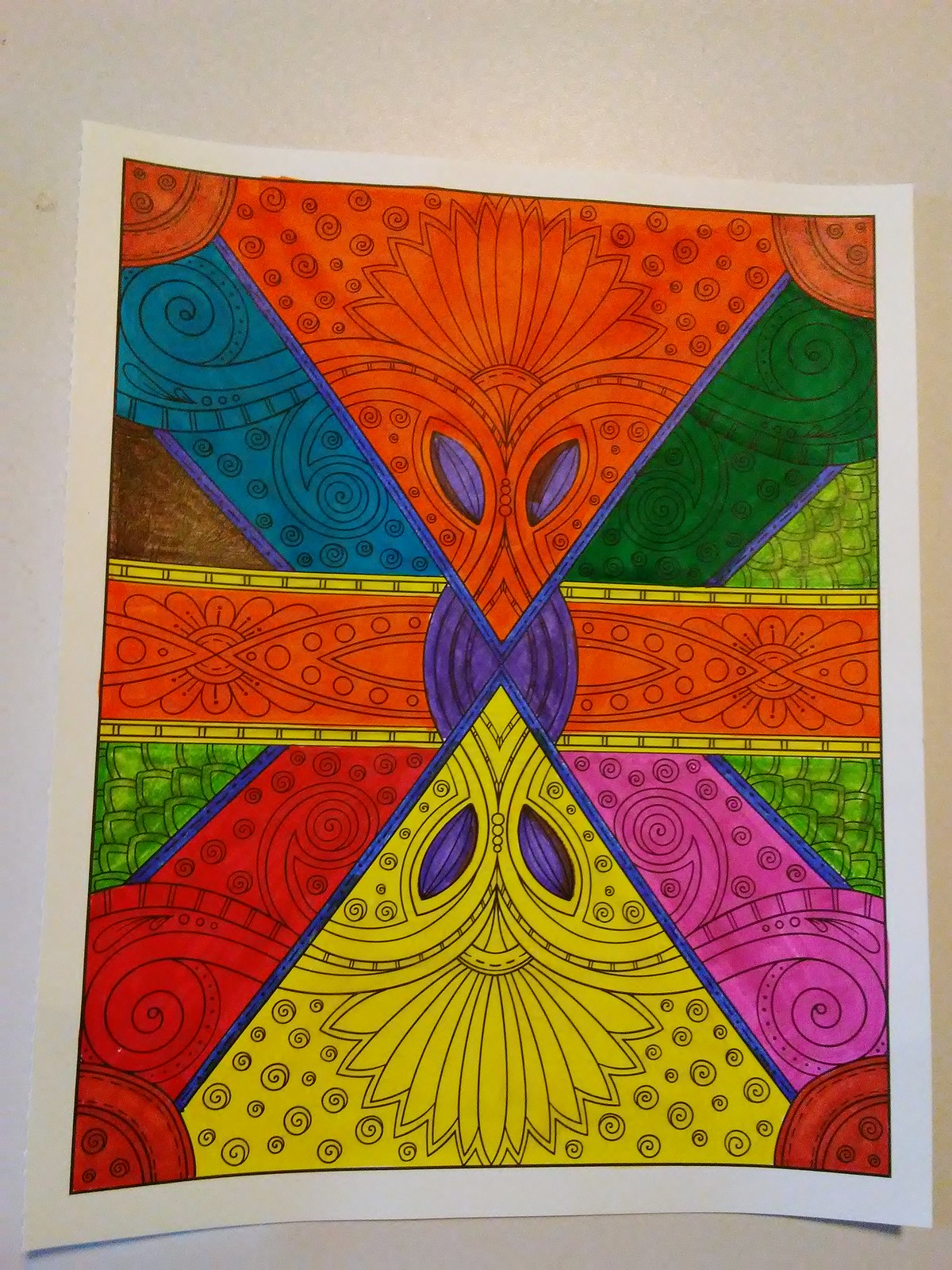In this photograph, we see a meticulously colored page from a coloring book, resting on a light gray or white countertop. The original drawing, executed in black ink, features an intricate, swirly floral design with somewhat psychedelic elements. These include fan-like leaves, spirals, and flower-like forms, as well as geometric shapes such as curves, pyramids, and partial ovals. The design radiates from a central, purple-colored portion, with purple outlining details emphasizing the center.

Color has been applied vibrantly across the design: the top section is filled with orange, creating a striking visual impact, while the corners are accented with brown and red hues. Sections emanating from the center include a spectrum of colors such as turquoise, dark green, red, and neon pink. The bottom section is primarily yellow, with green and brown providing additional contrast on the outer left and right sides.

The overall design is anchored around what appears to be V and X shapes, creating a dynamic, almost symmetrical pattern. The "V" shapes extend both upward and downward, with the upward V outlined in orange and featuring shapes akin to a masquerade mask with almond-shaped, purple "eyes." The horizontal segments of the X further diversify the color palette: the right is green and the left is blue at the top, transitioning into an orange stripe, while the lower left turns red and the lower right becomes pink.

Surrounding the main motifs are elements that resemble buttonholes within quarter circles, adding an additional layer of complexity with circular swirls and feather-like patterns. The blend of colors—orange, yellow, red, turquoise blue, purple, lime green, dark green, brown, and pink—creates a vivid, lively image that captures the eye and holds attention with its rich, multifaceted details.